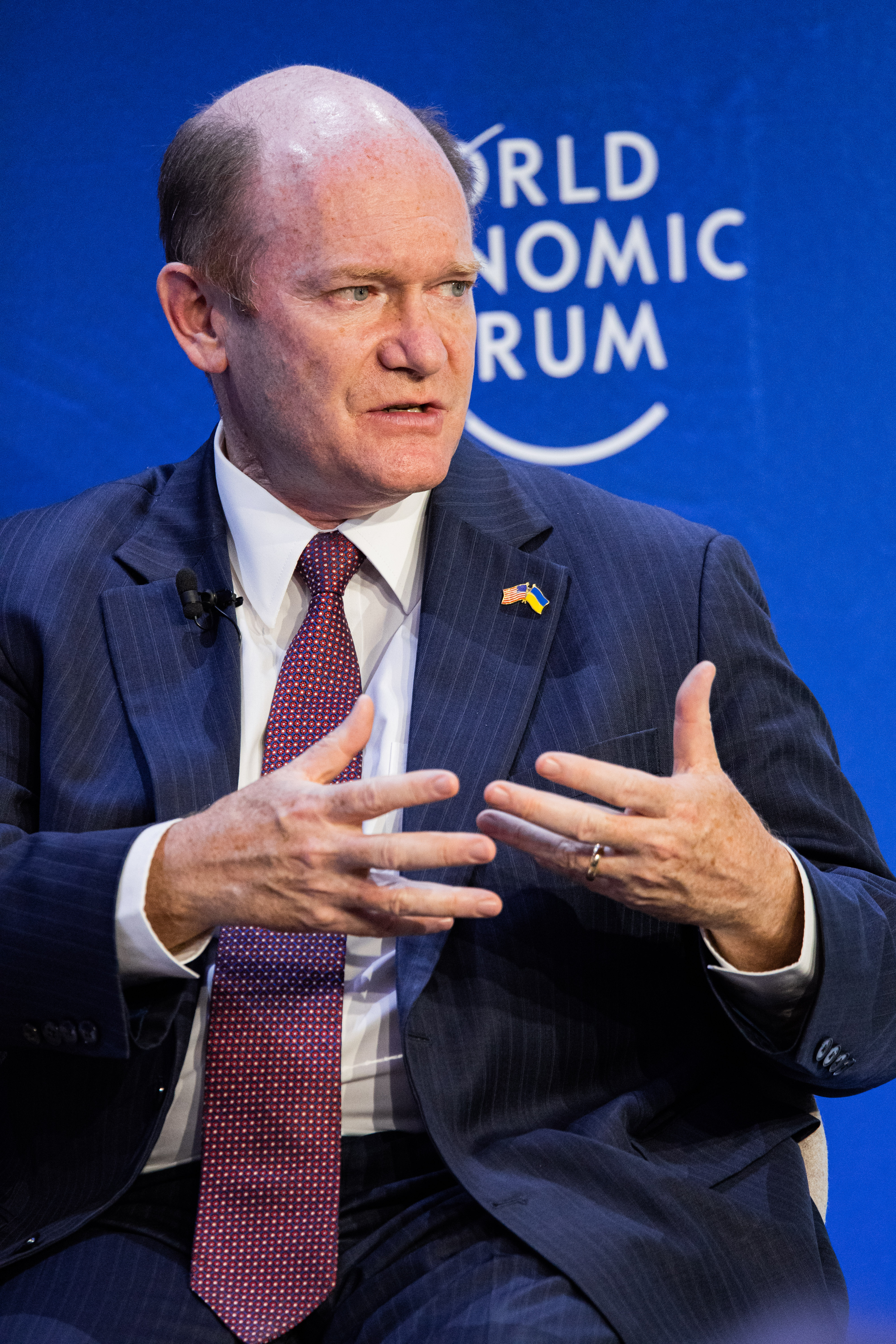The photograph captures a white male with brown hair, dressed in a blue pinstripe suit, who is seated and appears to be in the midst of a conversation or presentation. His suit features very thin white pinstripes, and he sports a red and navy blue tie with white dots over a white dress shirt. On his left lapel are two pins: one resembling the American flag and the other a blue and yellow striped flag. The man's head and hands are slightly turned to his left, as he appears to be engaging with someone off-frame in that direction. His hands are raised in front of him, and they appear somewhat wrinkled. The backdrop features a solid blue wall with the text "World Economic Forum" clearly visible in white letters, indicating the setting is likely a conference indoors. The overall color scheme includes blue, white, tan, brown, gray, maroon, and yellow.